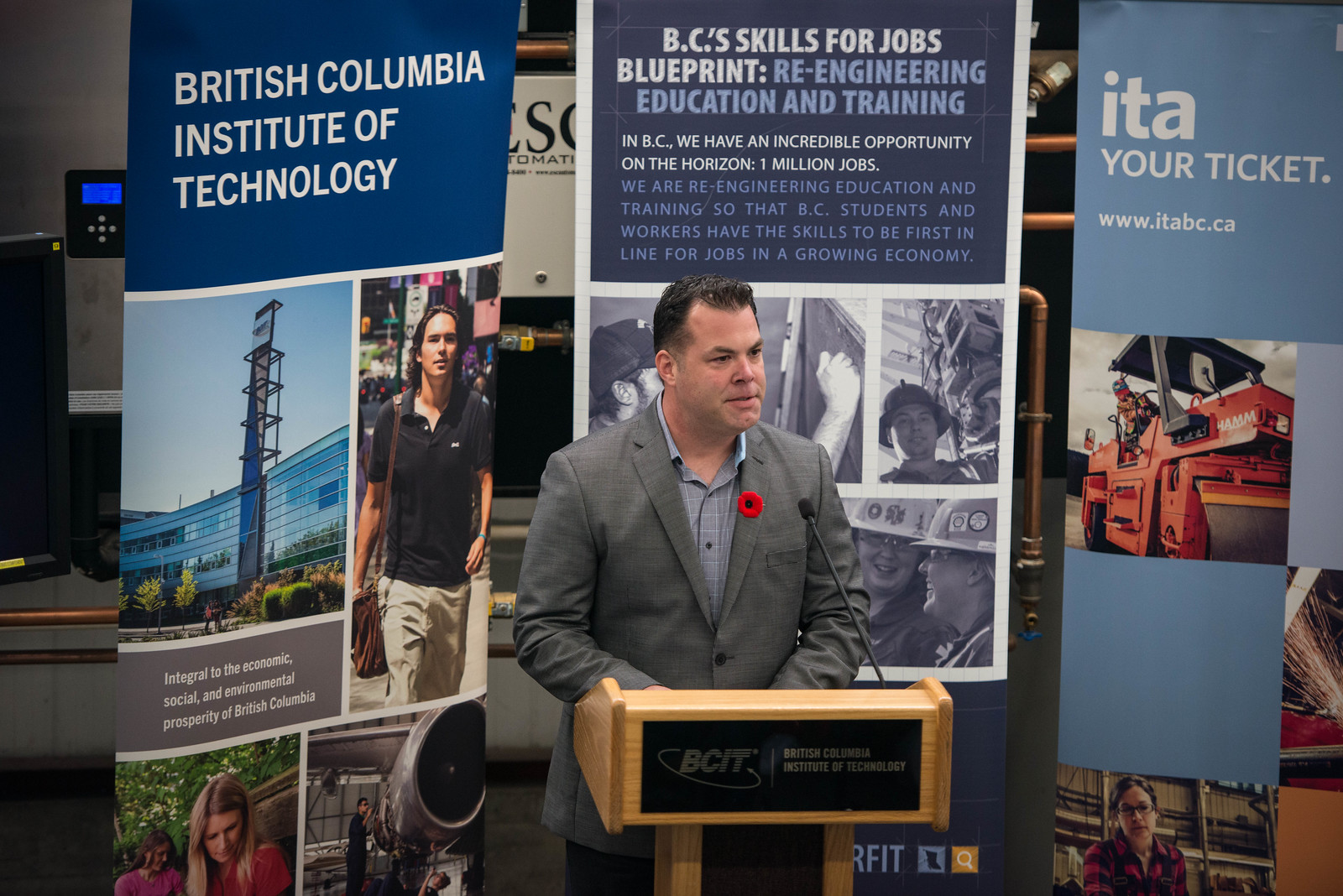In this photograph, a man in a gray suit and light blue shirt stands at a wooden podium with a black front displaying the BCIT logo, representing the British Columbia Institute of Technology. He has short, dark hair and is wearing a red pin or possibly a flower on his lapel. The background features three tall posters related to education and job skills in British Columbia. The first poster prominently bears the title "British Columbia Institute of Technology" and includes various pictures, including a crane, a confidently striding young man in work attire, a blonde woman in a pink shirt, and a uniformed person next to an airplane, suggesting the diverse training programs offered. The middle poster is titled "BC Skills for Jobs Blueprint" and has several black-and-white images, partially obscured by the speaker. It describes the goal of reengineering education and training to prepare students and workers for nearly one million job opportunities in a growing economy. The final poster reads "ITA Your Ticket" and includes the website "www.itabc.ca," as well as images of a man operating a bulldozer and another man wearing spectacles. The speaker’s impassioned expression suggests he is deeply engaged in his lecture on these educational and professional opportunities.